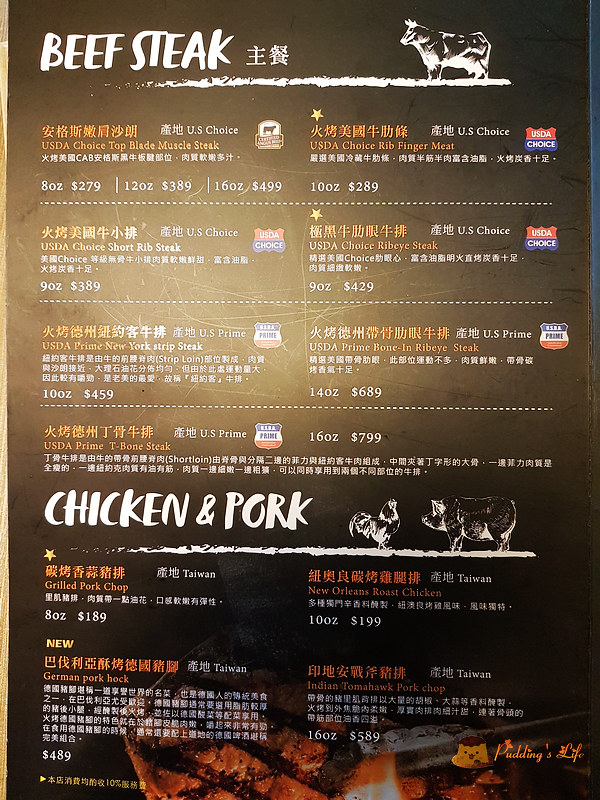This image features a detailed restaurant menu bordered by distinct designs on both sides. On the left, a rich brown wood-tone border frames the menu, while the right side showcases a gradient border transitioning from blue to black, perhaps influenced by the lighting. The menu itself is set against a brown background.

At the top left corner, the prominent white letters spell out "Beef Steak," accompanied by two characters in white that seem to be in an unfamiliar script. Below this title, a white line runs horizontally from near the word "Steak" towards the right edge of the menu. This line is jagged, resembling white grass, and it features a white silhouette of a bovine—likely a cow or bull—standing and looking to the left.

The menu highlights various USDA beef selections. The text is in yellow and white, with translations in at least one other language. Some of the featured items include USDA Choice Top Blade Muscle Steak and USDA Choice Ribbed Finger Meat. The prices, which are in a currency that is not immediately recognizable as American dollars, seem quite high, with entries like $279, $389, $499, $289, $389, $429, and $459.

Additionally, the menu lists USDA Prime T-Bone Steak priced at $799 for a 16-ounce portion. The bottom section of the menu mentions chicken and pork offerings, along with further details, though they are less prominently displayed.

In the bottom right corner, a cheerful note in yellow text reads "Pudding's Life," accompanied by a small yellow icon featuring what appears to be a head with a beak or mouth and red-brown hair. This playful addition adds a touch of whimsy to the otherwise formal menu.